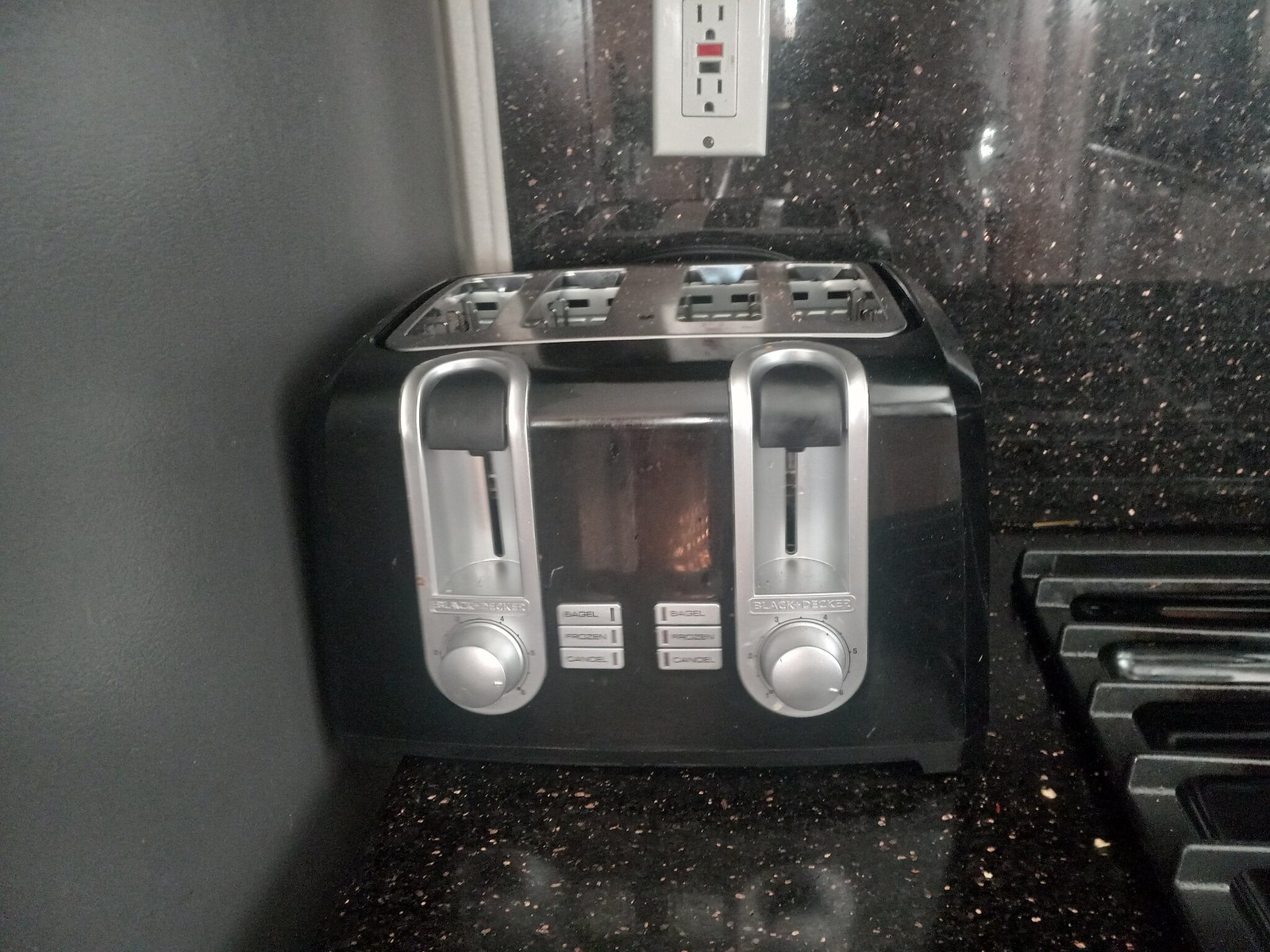This color photograph vividly captures the corner of a kitchen countertop, showcasing a high-end, four-slot toaster. The sleek toaster, primarily black with two silver oval control panels, has distinct features including two black levers for lowering bread, and silver knobs beneath for adjusting settings. Each side of the toaster is independently controlled, with three preset buttons per side—the top button on the right clearly labeled "Bagel." Positioned against a vibrant black granite countertop speckled with beige or white flecks, the toaster stands out under a silver outlet on the backsplash, which currently has no plugs inserted. To the right of the toaster, the edge of a black metal stove burner is visible. To the left, the scene is framed by a dark gray painted wall, adding a modern touch to the setting.